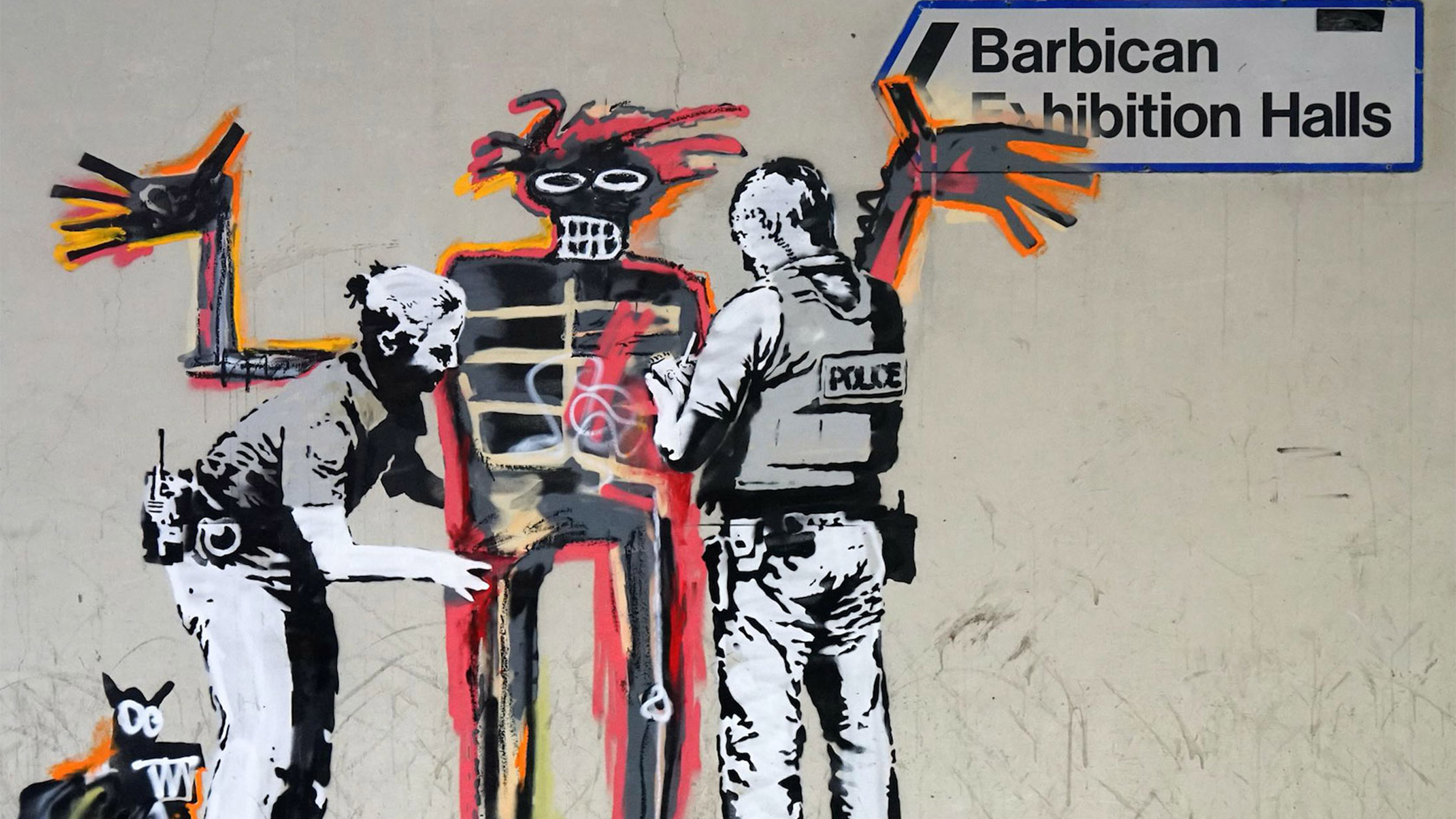In this detailed drawing set outdoors, the scene features two police officers, a woman and a man, against the backdrop of a wall with graffiti. The female officer, identifiable by her short hair tied in a bob and her short sleeve shirt and pants, is bending down to touch a graffiti painting of a distinctive skeleton. This skeleton, with outstretched arms and open hands, is framed in black with an orange border, has white eyes, a prominent set of teeth, and a head adorned with numerous red braids. Meanwhile, the male officer, donning a vest labeled "Police," stands to the right with his back slightly turned, diligently writing on a pad of paper. In the upper right corner of the image, the sign "Barbican Exhibition Halls" is prominently displayed against a cream background. Additional graffiti on the wall includes an image of a dog with white eyes and teeth situated in the bottom left corner. The intricate details of the skeleton, with its visible bones and muscles, add a monster-like appearance to the artwork, emphasizing the blend of art and surrealism in the scene.